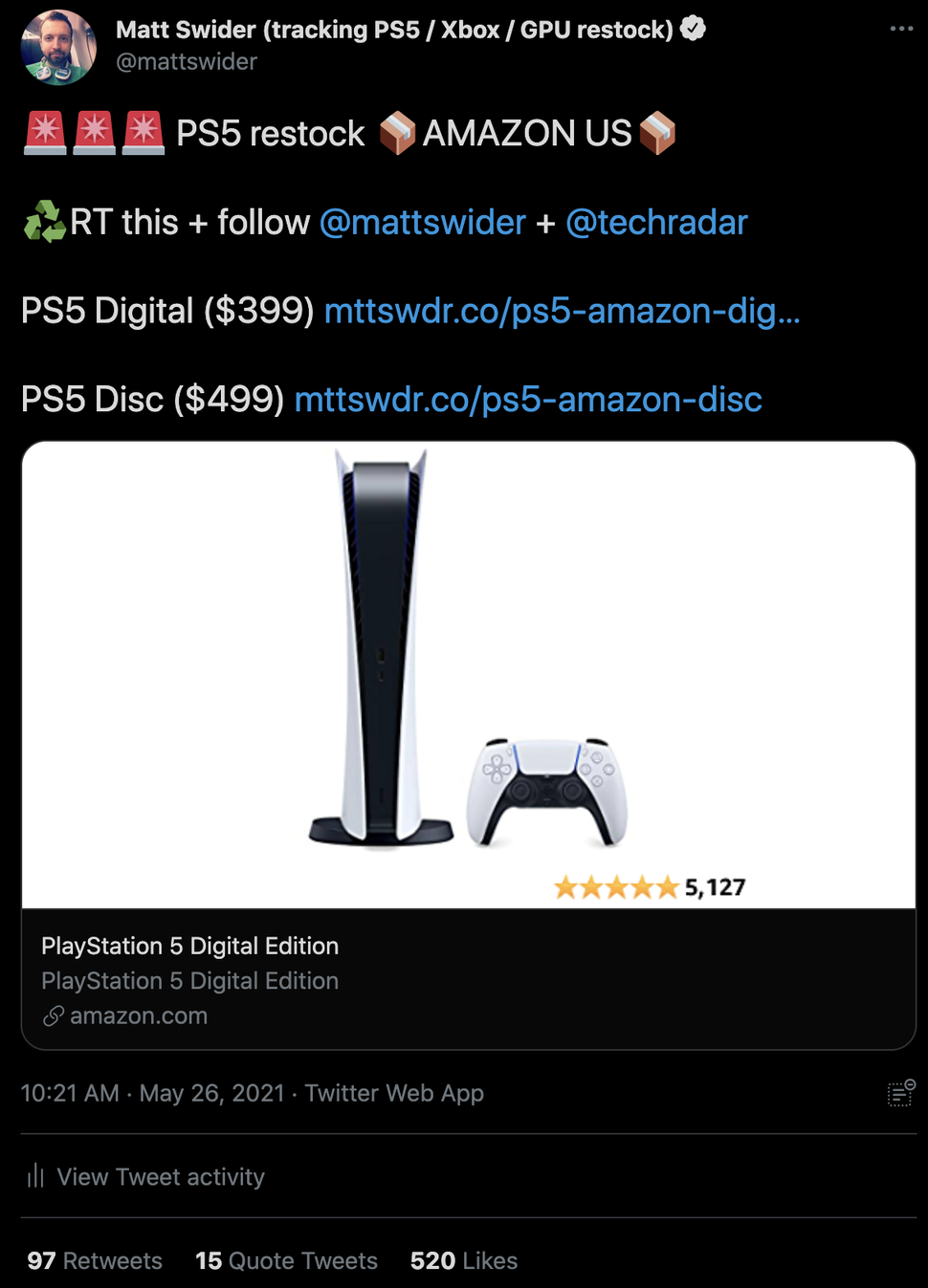**Screenshot of a Twitter Post in Dark Mode**

**Poster:** Matt Swider (Tracking PS5/Xbox/GPU Restock) ✅   
**Username:** @MattSwider

**Post Content:**  
🚨 PS5 restock 🚨  
📦 Amazon US shipping box 📦  
♻️ RT this + follow @MattSwider + @TechRadar ♻️  

**Details:**  
- **PS5 Digital Edition** for $399: [mttswdr.co/ps5-amazon-dig...](mttswdr.co/ps5-amazon-dig...)  
- **PS5 Disk Edition** for $499: [mttswdr.co/ps5-amazon-disk](mttswdr.co/ps5-amazon-disk)  

**Attached Image:**  
- A PlayStation 5 with a white case and a white controller.  
- Underneath, a rating of 5 stars based on 5,127 ratings.  

**Link Preview:**  
- **Amazon.com:** PlayStation 5 Digital Edition  

**Post Timestamp:**  
- **Date and Time:** May 26, 2021, at 10:21 AM  
- **Platform:** Twitter Web App  

**Interaction Metrics:**  
- **Retweets:** 97  
- **Quote Tweets:** 15  
- **Likes:** 520